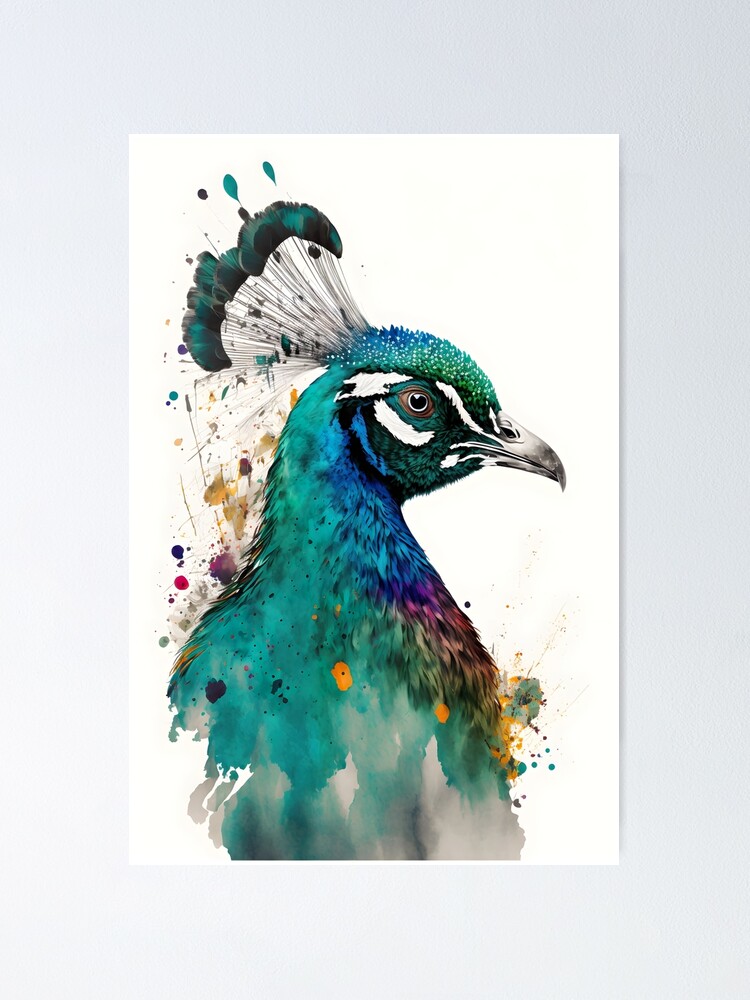The image portrays a detailed watercolor painting of a peacock principally showcasing its upper body, including the chest, neck, head, and crest. The artwork predominantly features shades of green-blue, with splashes of purple, pink, and yellow blending into the plumage. The peacock's head is realistically detailed with black pupils and white irises, and a gray beak, while its crest feathers exhibit a seafoam green interspersed with darker patches. The feathers on the breast include hints of red, orange, and yellow, adding to the vibrant palette.

The background is stark white, resting upon a gray surface or wall, suggesting it might be a print reproduction rather than a photographed piece on canvas or paper. The dimensions of the artwork are roughly twice as tall as it is wide, giving it a vertical emphasis. The intricate details are most pronounced in the neck and head, with the watercolor technique allowing the rest of the body to gradually fade out into a softer, blurred mixture of colors, creating a beautiful contrast between the sharp and muted elements of the painting. The overall composition highlights the elegance and vividness of the peacock while maintaining a modern and minimalist presentation.